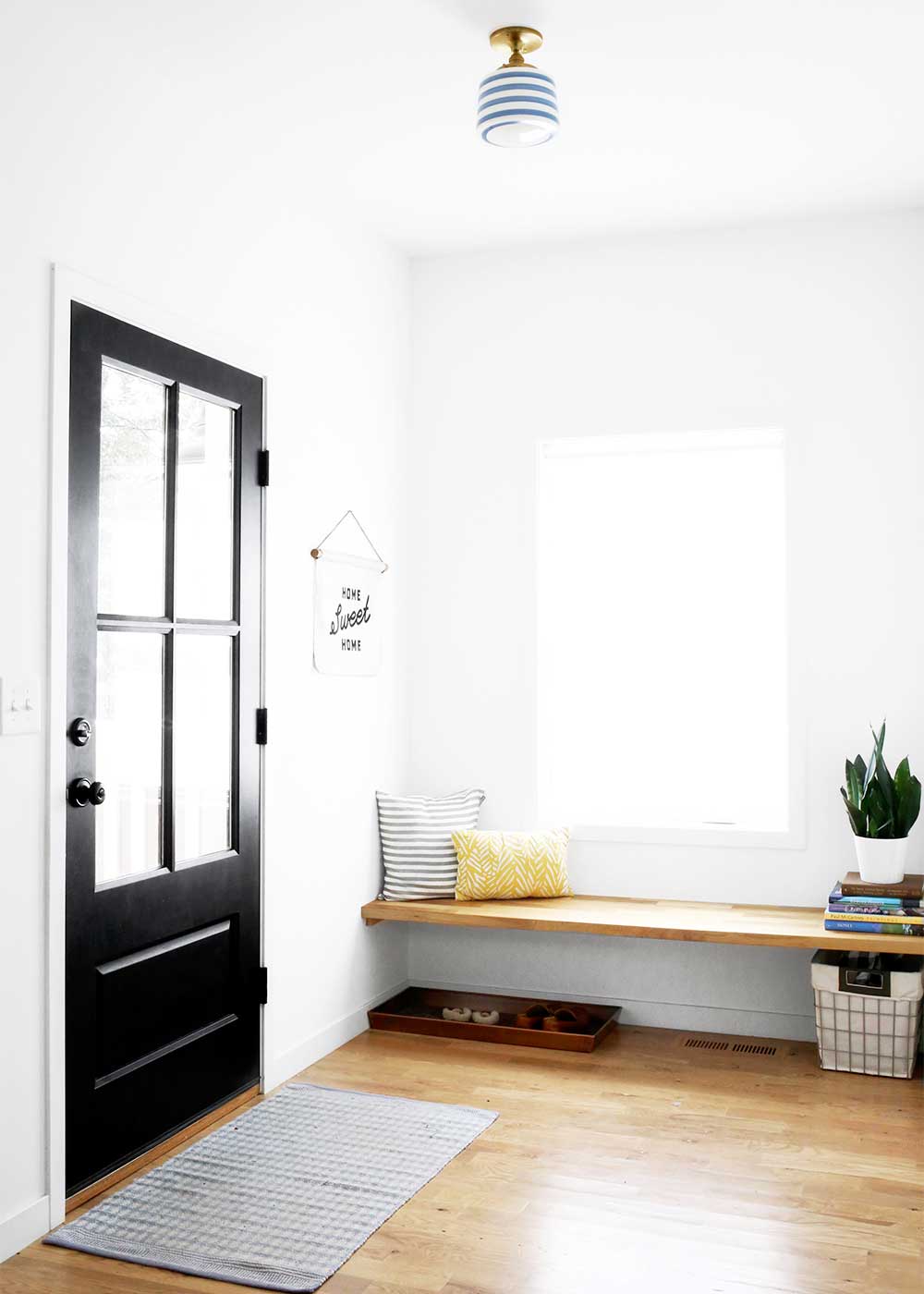This image portrays a bright, white entryway of a home with a contrasting black entry door featuring four rectangular glass panes. The flooring is wooden, and a wood bench is situated against the wall, adorned with a white and gray striped pillow, a yellow pillow, a few books, and a green plant in a planter. Below the bench, there is a shoe rack and a visible heating duct vent. To the right of the door, there’s a white light switch cover, while to the left, a white wall hanging with "Home Sweet Home" written in black lettering adds a welcoming touch. Covering the window in the door is a blind and placed in front of the door is a gray and white checked rug.